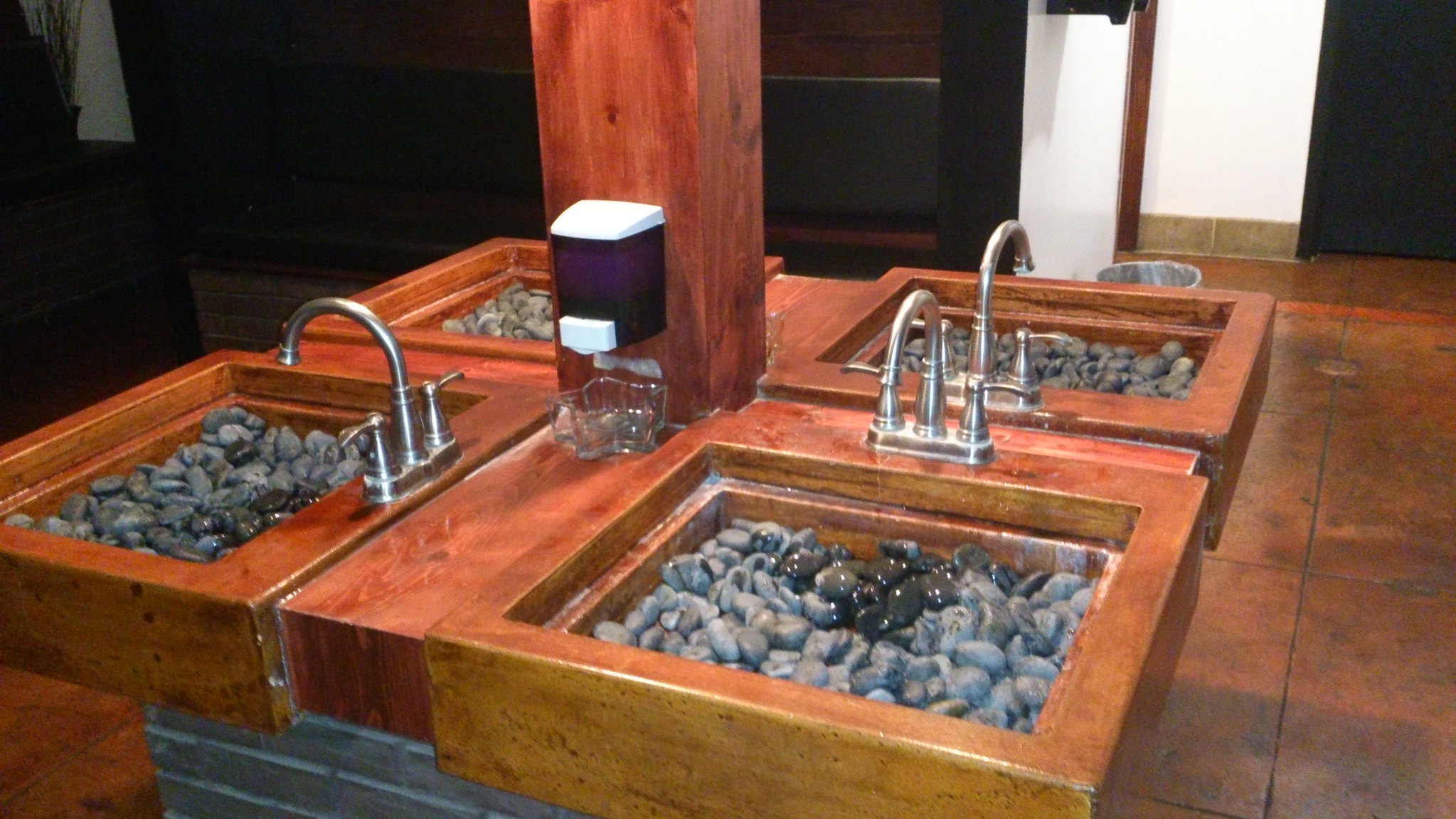The image depicts a uniquely designed public wash station featuring four wooden sinks with basins filled with gray river rocks, set up around a central wooden pillar. Each sink faces a different direction, and the faucets are curved and made of nickel, with separate handles for hot and cold water. The central pillar, which appears to be made of a russet-toned wood, supports two plastic soap dispensers accompanied by star-shaped clear bowls beneath them to catch any drips. The floor is covered with large terracotta Salteo tiles, complementing the earthy tones of the wash station. In the background, a silver metal trash can can be seen near the entrance or exit. The overall design includes a combination of two-tone wood and gray bricks, adding to the sophisticated and abstract aesthetic of the space.